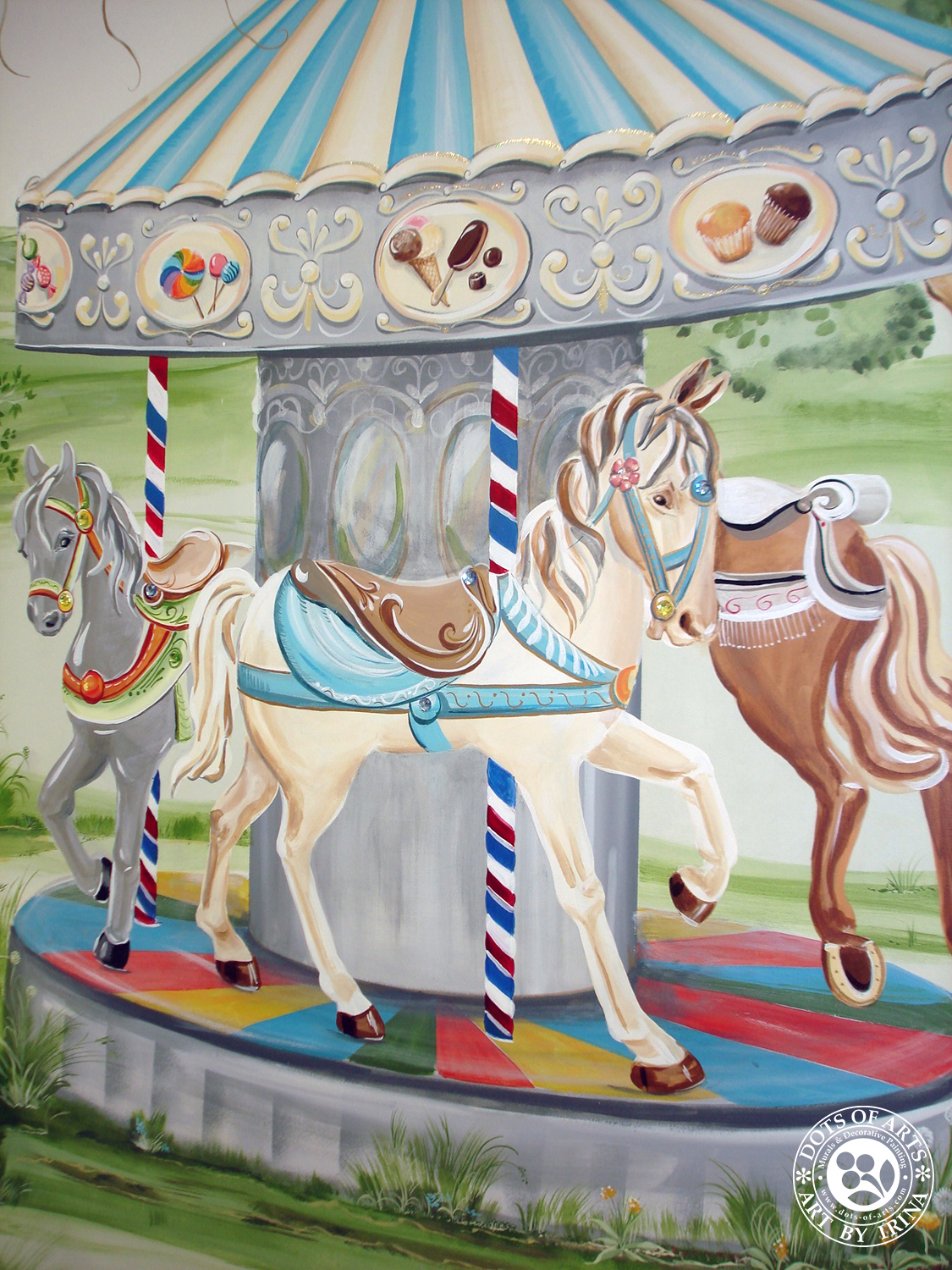This detailed illustration portrays a carousel in a vibrant, painted style reminiscent of a CGI or hand-drawn artwork. Dominating the top portion is the carousel's roof, featuring alternating blue and white stripes in pie-shaped sections. Below the roof, there's a decorative gray band adorned with intricate white designs and round emblems depicting various sweets such as cupcakes, ice cream, popsicles, lollipops, and candies.

In the central focus, three distinct horses are mounted on poles styled like barbershop poles, with diagonal red, white, and blue stripes. The foremost horse is white, equipped with a brown saddle over a blue blanket, and a matching blue harness. Positioned behind it is a gray horse, facing slightly forward and adorned with an orange, green, and brown saddle ensemble including a harness. To the right, only the hindquarters of a brown horse are visible, featuring a saddle and harness in shades of white, gray, and black.

The carousel rides on a gray base, with its floor divided into multi-colored, pie-shaped sections of red, yellow, blue, and green. The background hints at a natural setting with grass extending from the bottom left to the right of the image. Concluding the scene, a round, white emblem is noticeably placed in the bottom right-hand corner. The overall aesthetic captures a whimsical and nostalgic amusement park atmosphere.